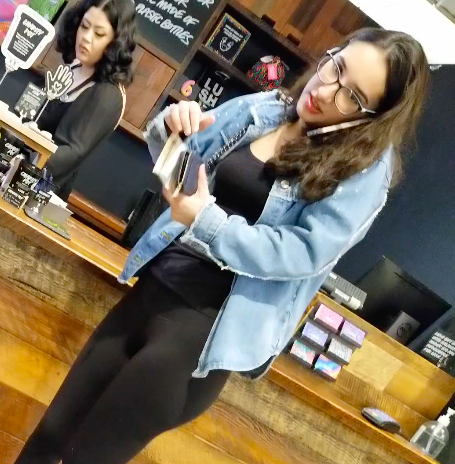In the image, we observe two females in what appears to be a store or cafe setting. The central figure is a Caucasian woman with long black hair and black-rimmed glasses. She is engrossed in her gray phone while fidgeting with her wallet and purse. She's dressed in a bluish jean shirt over a black top, paired with black fitted pants. 

Behind the counter stands another woman, who appears to have Asian features. She has dark curly hair and is wearing a black sleeved top. 

The scene features a brown wooden table beside the central woman, and a side wall adorned with a few cards. To the right, there is a debit machine and a clear bottle with a white pump, likely hand sanitizer. The backdrop on the right side of the wall is blue, while the rear wall behind the shelving unit is a rich brown hue. The shelving is gray, and a black chalkboard with white lettering reads "plastic bottles." A small white outline of a hand against a black background is mounted on a stick nearby.